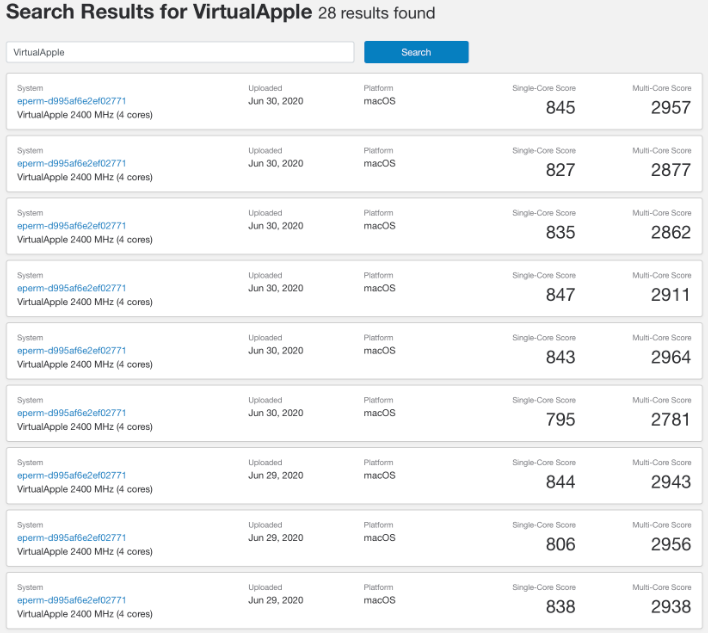This image is a detailed screenshot of a website, specifically displaying search results for "VirtualApple." The webpage has a very light gray background. At the top left corner, in bold black font, the text reads "Search results for VirtualApple," with the words "Virtual" and "Apple" combined into one word beginning with a capital "V" and "A." Adjacent to this, in a much smaller font, it states "28 results found."

Below this title, there is a search box, which is a long rectangular field. To the right of this search box is a blue rectangle serving as the search button, with the word "Search" displayed in white in its center.

Following these elements, there are nine rows of white rectangular boxes spread across the width of the page. Each of these boxes follows the same format and contains intricate details. At the top of each white box, the word “System” is written in extremely small gray font. Below this, there is what looks like a file name in blue text, such as "Eperm" followed by a dash and a long string of letters and numbers. Beneath this blue text, it says "VirtualApple, 2400 MHz" with "four cores" mentioned in parentheses.

Every row contains four columns of data. These columns display the date, the platform, the single-core score, and the multi-core score, with specific numbers and information pertaining to each column. This consistent format is maintained across all nine rows.